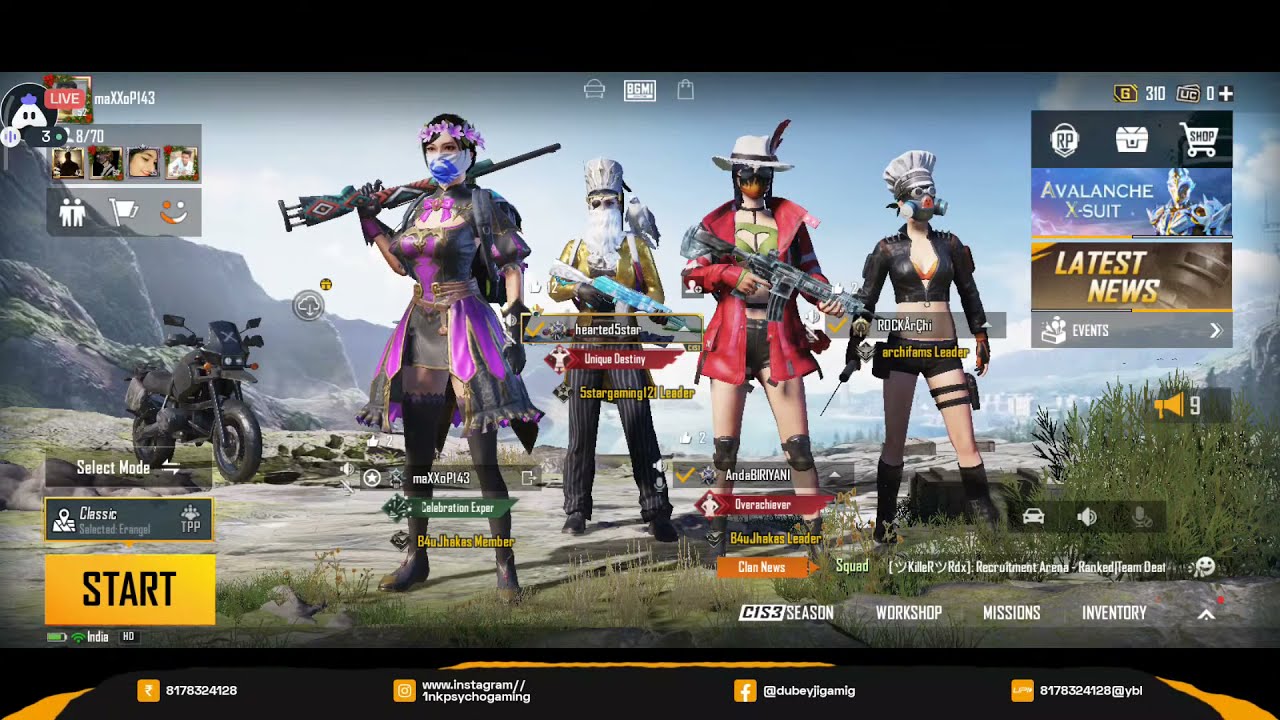This detailed screenshot of a lively video game interface features four central characters, each uniquely attired and armed, standing in a natural setting with hills, mountains, and trees in the background. On the left, a female character in a black suit with a short skirt, adorned with purple banners, sports a white and blue mask and a ribbon of purple flowers in her hair, holding a gun over her shoulder. Behind her, an older male character with a long white beard wears a yellow shirt, black pants, and a white hat, gripping a white and light blue gun. The third character, a woman in a white hat with a feather, is dressed in a red vest, white suit, and black shorts, holding a gray gun pointed downward. The final character, also female, dons a white cook's cap, a gray gas mask, a black open coat revealing a purple bra, black shorts, and a black holster on her right leg, holding a spiked object in her left hand. 

In-game details crowd the frame: the bottom left icon is an orange "Start" button, with "Classic" above it and "Select Mode" further up. The upper right corner displays "310", a zero, a plus sign, and various game icons like a shopping cart and "RP", along with "Avalanche Axe Suit", "Latest News", "Events", and a loudspeaker symbol next to the number 9. The lower section features labels such as "C1S3 Season", "Workshop Missions", "Inventory", and "Clans News". The upper left corner shows a red "Live" icon, the numbers "8-710", four pictures beneath it, and a pictogram of two people and a flag. Under each character, names like "Hearted", "S-S-T-A-R", "Rocker Girl", "Anda Biryani", and "My XXOP143" are displayed along with their levels and leader status. A black or dark gray motorcycle is visible to the left of the characters, adding to the dynamic and busy game layout.